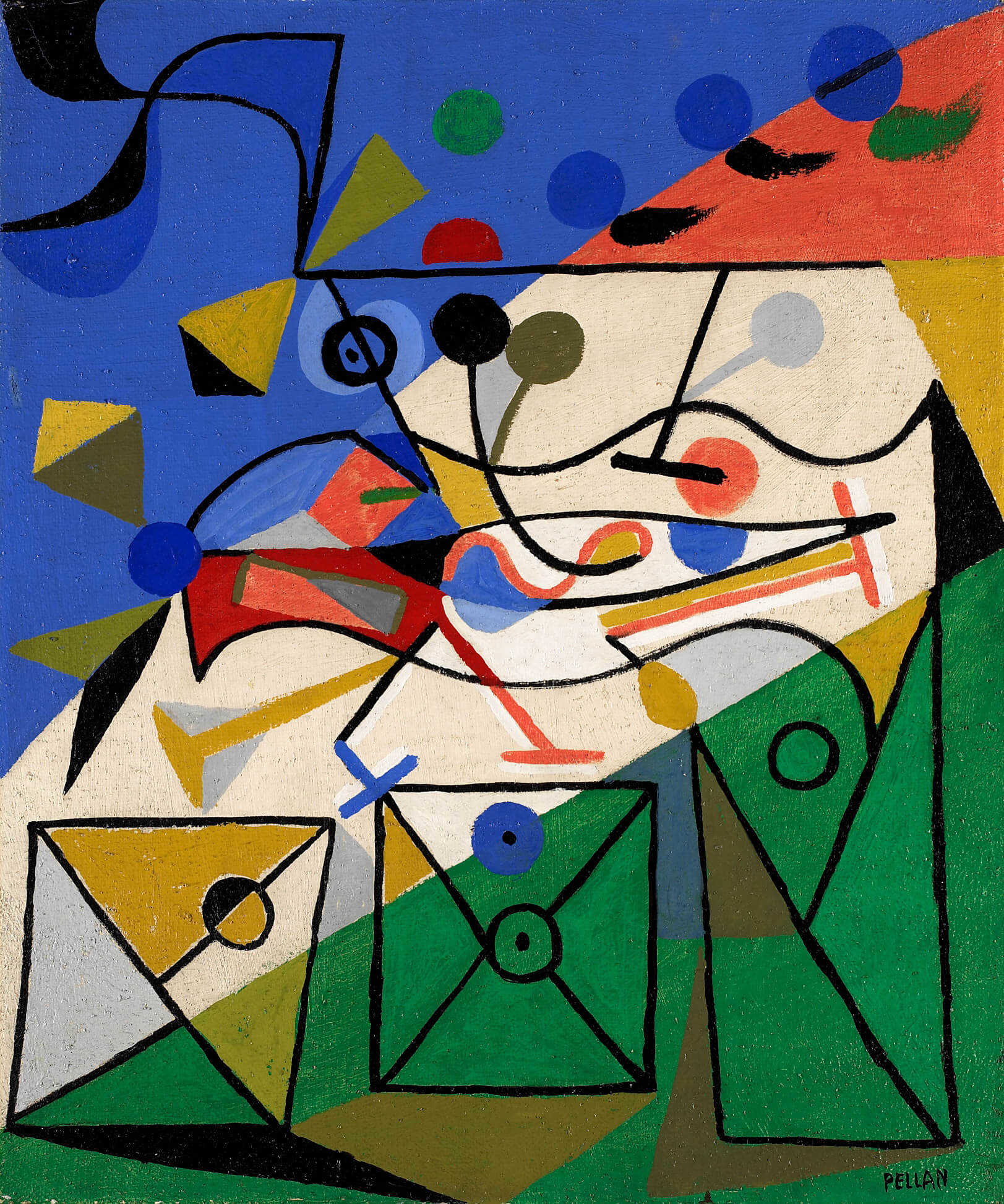This is an abstract, Picasso-style painting by the artist Pellen, as noted by the small black signature in the bottom-right corner. The painting is diagonally divided into three color sections: blue at the top left, off-white or beige in the middle, and green at the bottom. The top-left corner features a large blue triangle dominating the area, filled with various geometric shapes such as yellow rhombuses, diamonds, red semicircles, and a green circle. A continuous black line runs along the border of the painting, adding to its structural composition. 

At the center of the painting, a complex abstract shape draws attention with its white face, red tail, and a leg that appears to be both red and blue, bearing semblance to a bird or another unidentifiable figure. This central figure is layered with numerous shapes and patterns, including kite shapes, circles, half-circles, and different colored lines resembling nails or golf tees in red, blue, white, and black. 

The bottom-right section, which is mostly green, contains what resemble stained glass shapes or boxes resembling letters and envelopes with various folding patterns and circles in green, black, yellow, white, and black. The upper-right area features blue circles and black and green brushstrokes that complement the painting's overall abstract and geometric design.